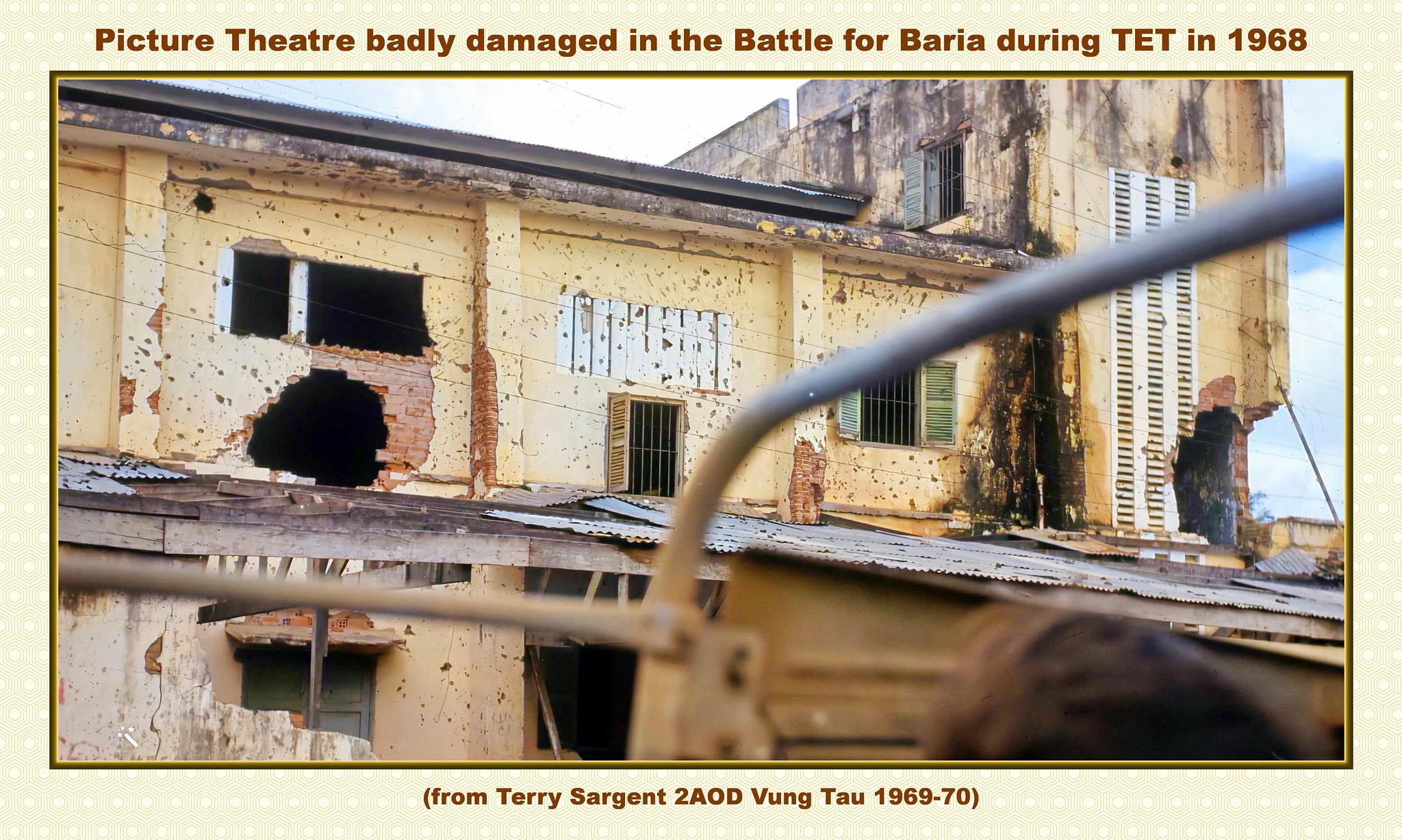The image depicts the exterior of a decrepit and battle-scarred building, identified by an inscription at the top as a public theater severely damaged during the Battle for Baria in the Tet Offensive of 1968. The structure, seemingly on the verge of collapse, exhibits significant wear and tear with multiple chunks missing from its facade. Its dirt-colored walls are peppered with darkened patches, indicative of the intense conflict it endured. The vantage point appears to be from a moderate distance, capturing the full extent of the building's dilapidation and giving a somber testament to its historical significance.